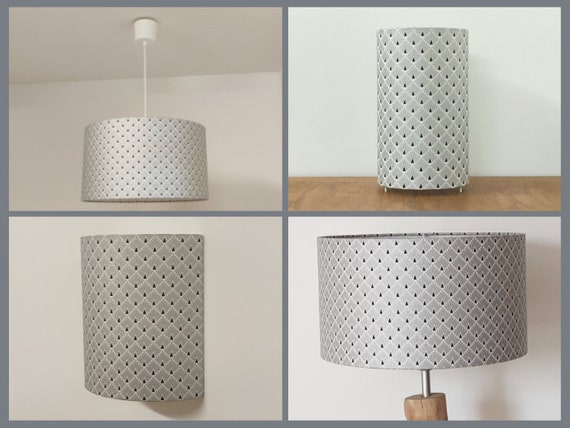This image presents a meticulously arranged grid of four different styles of lamps, each against a light gray or beige backdrop, divided by dark gray gutters. The top left quadrant features a ceiling lamp suspended by a whitish hanger, while the top right shows a narrow, vertical standing lamp. In the bottom left quadrant is a wall sconce, and the bottom right showcases a classic table lamp resting on a brown wooden table against a light gray wall.

All lamps share identical, intricate lampshades composed of a papery material adorned with a diamond grid pattern. The diamond shapes are formed by criss-crossing white lines, with a small hole drilled at every intersection, creating a dotted appearance. Each diamond also features a black teardrop shape at its bottom. The cohesive design, varied lamp styles, and uniform aesthetic against the subtle background combine to offer a detailed, visually appealing display of lighting fixtures.